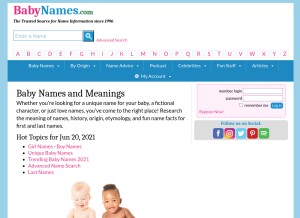The image features the homepage of BabyNames.com. The logo is prominently displayed in the upper left corner with "Baby" in large, pink letters, followed by "Names" in blue letters and ".com" in black. Below the logo, there is fine print in black that is difficult to read.

A search bar is positioned beneath, outlined in blue with a blue search icon. Next to it, "Advanced Search" is written in pink. Directly below the search bar is the alphabet, displayed in pink letters.

A blue navigation bar appears under the alphabet, with the first clickable category titled "Baby Names." There is white text below the navigation bar that reads: "Baby Names and Meanings: Whether you’re looking for a unique name for your baby, a fictional character, or just exploring names, you’ve come to the right place. Research the history, origin, and meaning of a wide range of names." The rest of this text is not clearly visible.

The section titled "Hot Topics for June 20th, 2021" is written in black, featuring a list of items denoted by black bullets and pink text.

Towards the right, there is a pink box where users can enter information, possibly a password. This section also contains icons for various social media platforms, including Facebook, Instagram, Twitter, Reddit, and WhatsApp.